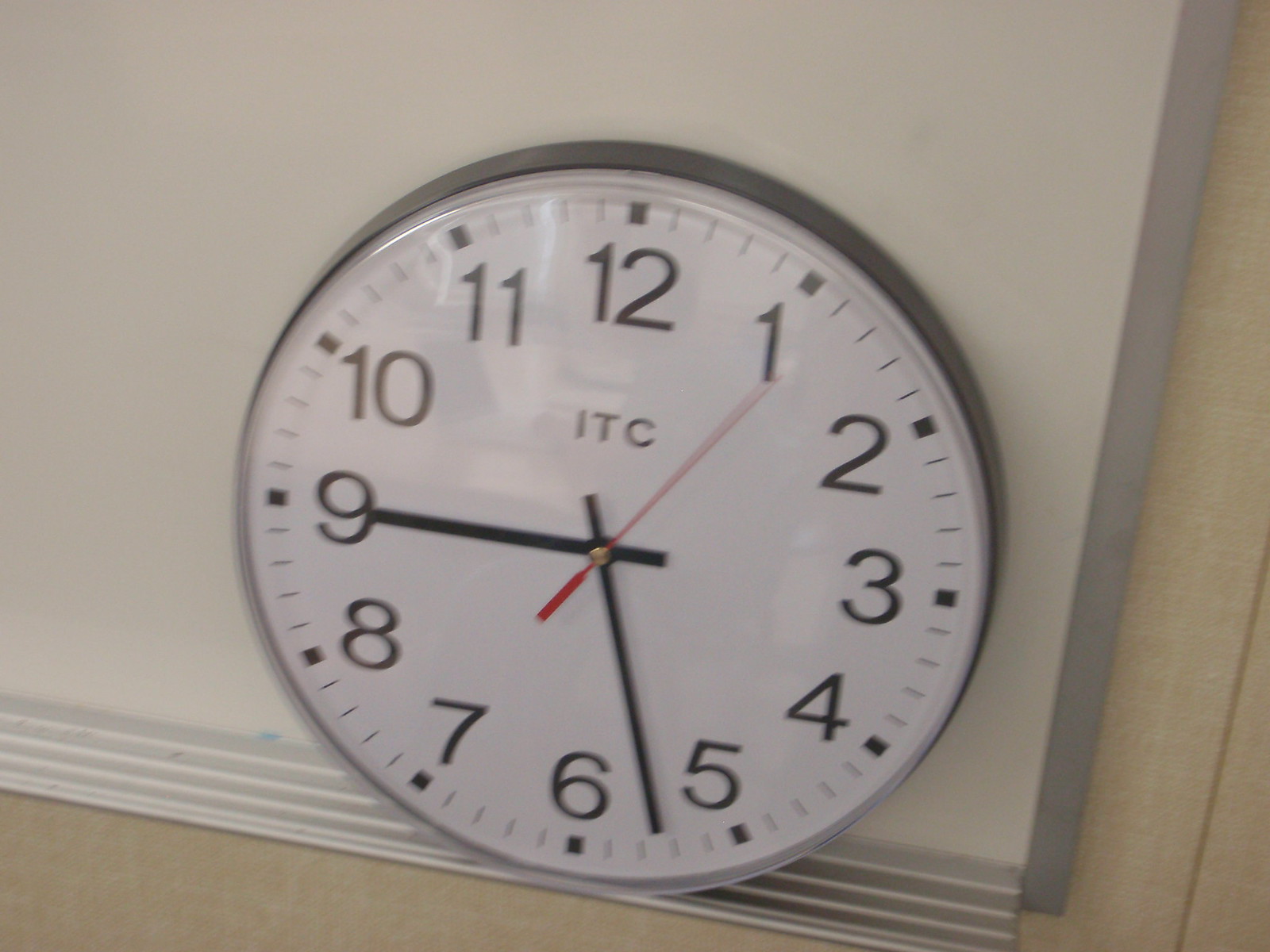The digital photograph taken indoors features a classroom-like environment. Dominating the right and bottom portions of the image, there is a tannish colored wall. A significant portion of the frame, spanning from the upper left to near the bottom right, is occupied by a whiteboard with a gray strip on the right edge and a larger silver strip at the bottom designed for holding markers. Placed on the far right side of the whiteboard’s bottom ledge is an analog clock with a black rim. The clock face is white, displaying black numerals from 1 to 12 in their correct positions. The clock's hands, including the hour and minute hands, are black, while the second hand is red. The time indicated on the clock reads around 9:27 with the second hand at 7 seconds. Additionally, the initials "ITC" are printed in black beneath the 12 and above the clock hands' center.